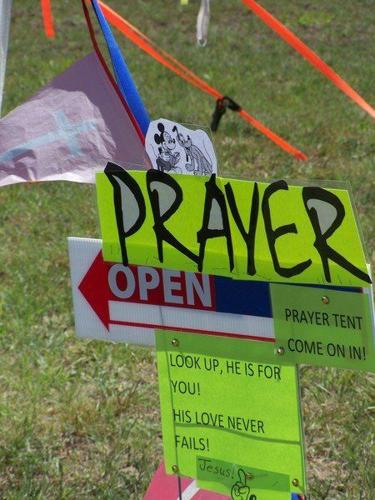This vertically oriented photograph captures a vibrant scene set outdoors, presumably during the day, featuring a handmade sign planted in the ground amidst a patch of green grass. The top of the sign showcases a black-and-white illustration of Mickey Mouse and Pluto, adding a playful touch. Attached to the existing sign (originally an open house sign, now repurposed), are several neon green and yellow paper sheets with black text, secured with tape, and an open house sign with a red arrow pointing left.

The first neon green sheet says "Prayer" in black text, with the inner loops of the letters highlighted in white for emphasis. Below it, another green paper reads "Prayer Tent, Come on in." Further down, a third green piece of paper bears the inspiring message, "Look up, He is for you. His love never fails. Jesus," along with a hand-drawn pointing hand. There's an additional white sign with a red arrow that reads "Open."

In the background, a small red flag with a white cross, possibly part of the prayer tent, and some orange-red straps are visible, adding to the detail of the setting.